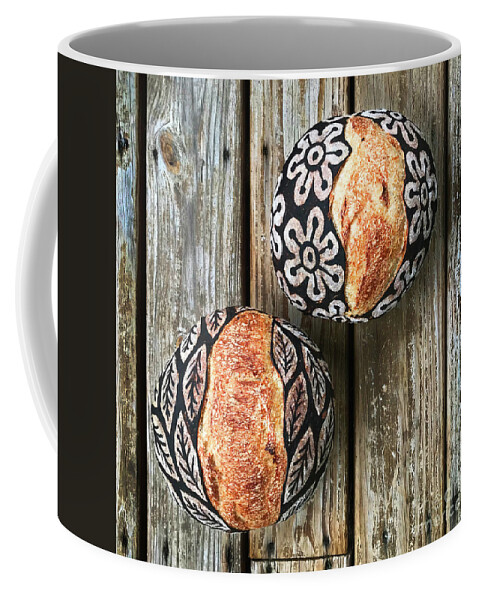This image features a close-up of a black coffee mug with a white handle and rim, set against a white background. The central focus is the detailed photograph wrapped around the mug, depicting two intricately designed homemade loaves of bread in a rounded boule shape. The loaves sit on a rustic, weathered wooden tabletop where you can see the spaces between the planks. Each loaf is artistically decorated: the upper loaf on the right showcases an abstract flower design, featuring white petals surrounding black spokes with dots at their ends, emanating from a central dot. The lower loaf on the left is adorned with a leaf design; white leaves with black veins stand out against a black background. The slashing on the bread is a traditional brown in the middle, while the sides are painted black, possibly with sesame. Both loaves are angled slightly, adding to the visual appeal and emphasizing the meticulous craftsmanship involved.